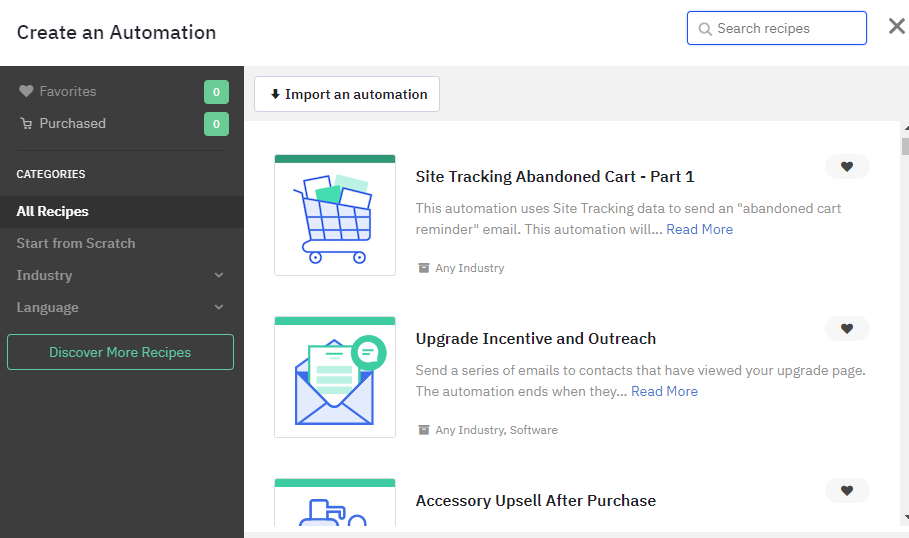In the top left corner of the image, there is a label that reads "Creates in Automation." On the top right, within a search bar area outlined in blue, it says "Search Recipes," accompanied by an 'X' icon to the right of the search bar. Moving to the far left, a column of categories is visible. The first category, labeled "Favorites," is represented by a heart icon to its left. Below is "Purchased," denoted by a shopping cart icon. Following this is the heading "Categories" itself, which is succeeded by several specific categories listed as: "All Recipes," "Start from Scratch," "Industry," "Language," and a rectangular shaped button labeled "Discover More Recipes."

Centrally positioned and slightly higher within the image, the word "Import in Automation" is prominently displayed. Beneath this header, a section titled "Site Tracking Abandoned Cart Part One" is shown. It explains that the automation leverages site tracking data to dispatch an abandoned cart reminder email. Below this, there is another section labeled "Upgrade Incentive and Outreach," which outlines a series of emails directed to contacts who have visited the upgrade page. The automation sequence concludes with a trailing "Read more" link, presented in blue text, indicating additional information to follow.